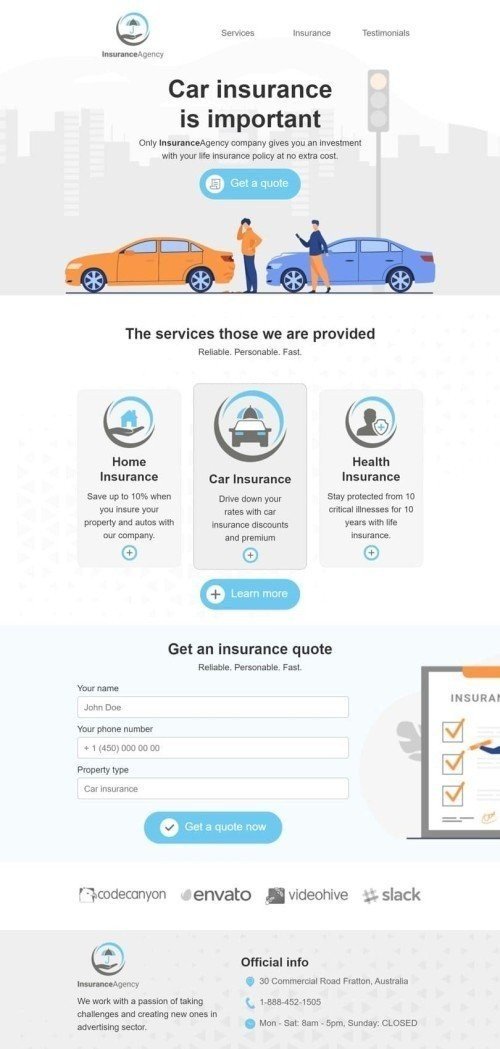This is a portrait-oriented screenshot from a cell phone displaying a car insurance app or website. The image, roughly the size of a cell phone screen, lacks defined borders. 

At the top, there's a logo resembling a circle with a hand holding up an umbrella, accompanied by menu options labeled "Services," "Insurance," and "Testimonials." The company's name beneath the logo is too small to discern. Below this, a box features a grayed-out cityscape background and a black header that reads, "Car Insurance is Important." Additional text (illegible in the photo) follows, along with a blue oval button marked "Get a Quote."

In the foreground, two cartoon cars, one orange and one blue, are depicted with people standing in front of them and a grayed-out stoplight. The lower section of the image primarily shows a white background, except at the bottom where it mentions provided services: "Home Insurance," "Car Insurance," and "Health Insurance," each with corresponding icons. "Car Insurance" is visibly selected.

Below, a section headed "Get an Insurance Quote" includes input boxes for entering a name, a "Get a Quote Now" button encapsulated in a blue oval with white text, and a white circle containing a black check mark. At the bottom, a gray box offers additional company information.